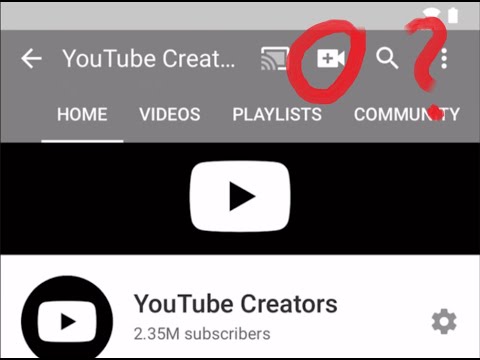The image is a detailed user interface layout, featuring several distinct sections and icons. At the very top, there is a light gray box containing two small white images. Below this, a darker gray box includes a left arrow and the text "YouTube Create." This section also houses four small icons: a screen with a radar-like symbol in the corner, a red circle around a camera, a magnifying glass, and a red question mark, accompanied by three white dots. 

Underneath these elements, a navigation menu displays the options "Home" (which is underlined), "Videos," "Playlists," and "Community." Below this menu, there is a black box inside which a white box with a black right arrow is positioned. Adjacent to this is another white box, which features a black circle containing a white box with a black right arrow and the text "YouTube Creators." This section also indicates the channel's subscriber count, 2.35 million, and includes a small gray cog icon on the right side. A black line runs horizontally across the bottom of the image, providing a clean division.